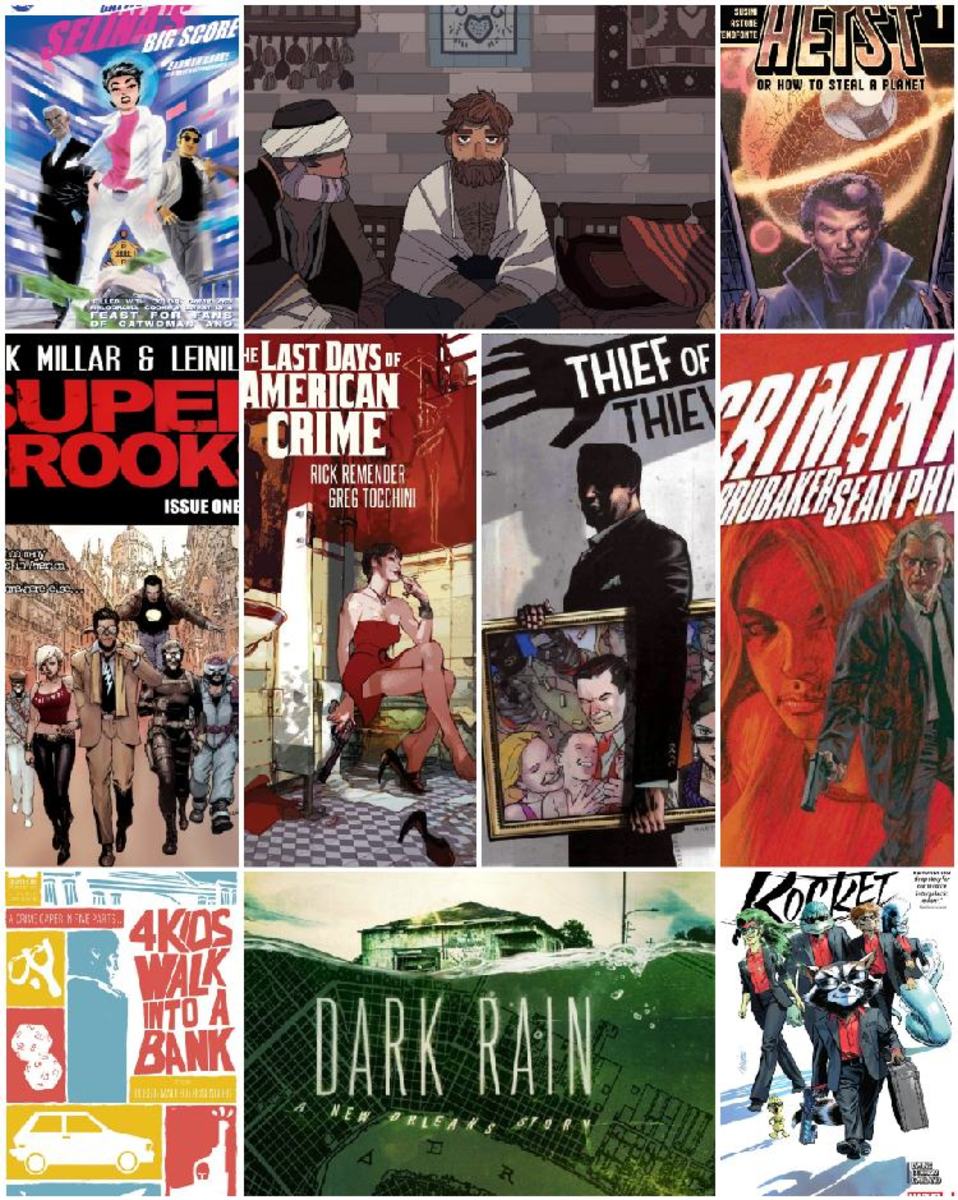This image is a detailed advertisement showcasing a variety of graphic novels, each illustrated with hand-drawn or painted artwork. The layout features three rows of images, with three panels in the top row, four in the middle row, and three in the bottom row.

In the top left panel, a graphic novel titled "Selina's Big Score" is depicted, featuring a woman clad in a white suit with a pink shirt underneath, flanked by two men. The central top panel portrays a serious-looking bearded man sitting beside another man wearing a turban-like hat against a brick wall backdrop. The top right panel advertises "Heist or How to Steal a Planet," showing a man with a planet resembling Saturn behind him, set against a background of space.

The middle row begins with "Super Crook," illustrating a team of superheroes following a man in a tan suit. Next to it, "The Last Days of American Crime" by Rick Remender and Greg Tuccini features a woman in a red dress sitting on a toilet, seemingly in a bathroom, possibly with blood around. The third panel in this row is "Thief of Thieves," which depicts a clean-cut man in a black suit and shadowed face holding a possibly stolen painting. The fourth middle panel is titled "Criminal," showing a distressed man in a gray suit holding a gun with a red-orange portrait of a woman in the background.

The bottom row commences with "Four Kids Walk Into a Bank," a vibrant and colorful montage using blue, red, and yellow themes, showcasing dice, cars, a slingshot, and guns. The central bottom panel titled "Dark Rain: A New Orleans Story" presents a house partially submerged in water, depicting the aftermath of a flood likely referencing Hurricane Katrina, with a map of the city visible in the green lower section. The final panel on the bottom right, titled "Rocket," features Rocket Raccoon from Guardians of the Galaxy, front and center, holding a briefcase along with three other animal-like characters behind him.